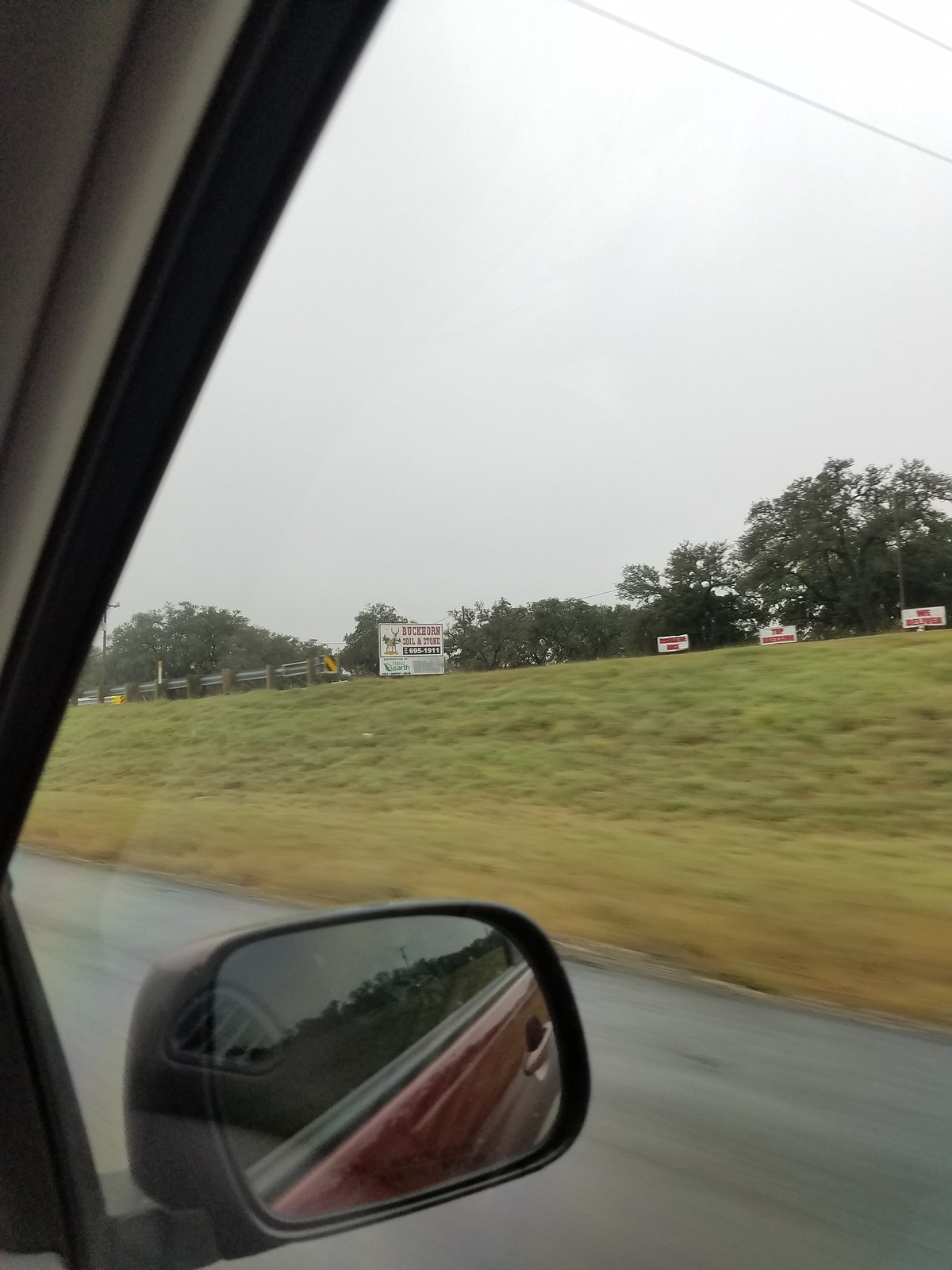An image captured from the passenger side of a moving car provides a glimpse into a rural setting. The reflection in the side-view mirror reveals that the car is an older model with a red exterior, as evidenced by the vintage door handle design. The window is rolled up, creating a faint glare that is visible in the photograph. The sense of motion is conveyed by the blurred appearance of the pavement beneath the vehicle. Across the street, a large billboard stands, though its message remains indiscernible due to the distance. Surrounding the billboard, an expanse of lush grass and trees dominates the landscape, emphasizing the rural environment. Three smaller signs accompany the billboard, but like the larger sign, their contents are too small to decipher.